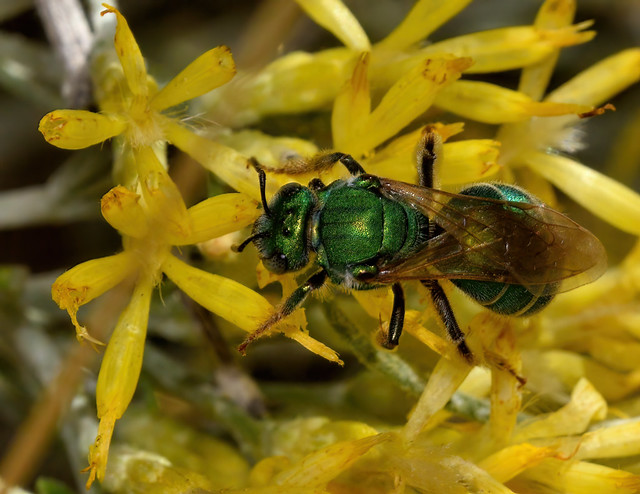This highly detailed, close-up image showcases a large green insect, likely a bee or cicada, perched on a vibrant bed of yellow flowers. The insect, positioned towards the center and slightly to the right of the frame, fascinatingly exhibits a metallic green body adorned with tiny hair-like features and fuzz. Its brilliant green color is accentuated by its black legs, black eyes, and two distinct black antennae. The insect’s wings are a transparent brown, neatly folded along its back. Its legs, with those on the left extending downward and those on the right appearing at the top of the image, add to the dynamic portrayal. The yellow flowers, with five-section petals, have browning or decayed tips and form the bright, detailed backdrop for the insect, making it the clear focal point of the photograph. The image is so sharply focused that even the minute details of both the insect and the flowers are vividly captured, highlighting the intricate beauty of nature up close.